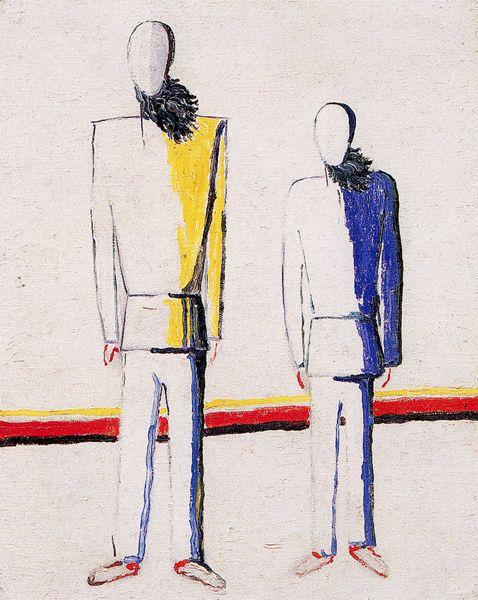This image portrays an artistic fashion design of two faceless sketches, set against a stark, blank background. The taller figure on the left, presumed male, is adorned in a unique tunic featuring yellow elements on the right side, complemented with a distinctive square jacket that boasts oversized shoulders and a fur-like collar or scarf. This outfit is rounded off with white pants and white shoes accented with red heels. Adjacent to him stands a shorter figure, presumed female, clad in a similar style tunic but with blue details on the left side extending down the sleeve. She also has something wrapped around her head and neck, accentuating the ensemble, which is completed with white attire and identical white shoes with red heels. The backdrop includes a horizontal stripe emblazoned in yellow, red, and black, adding a dash of color symbolism and cultural reference. Both figures feature beards, possibly artistically interpreted, blowing in the wind, standing stock-still, facing forward with their arms naturally resting at their sides, embodying simplicity and elegance.